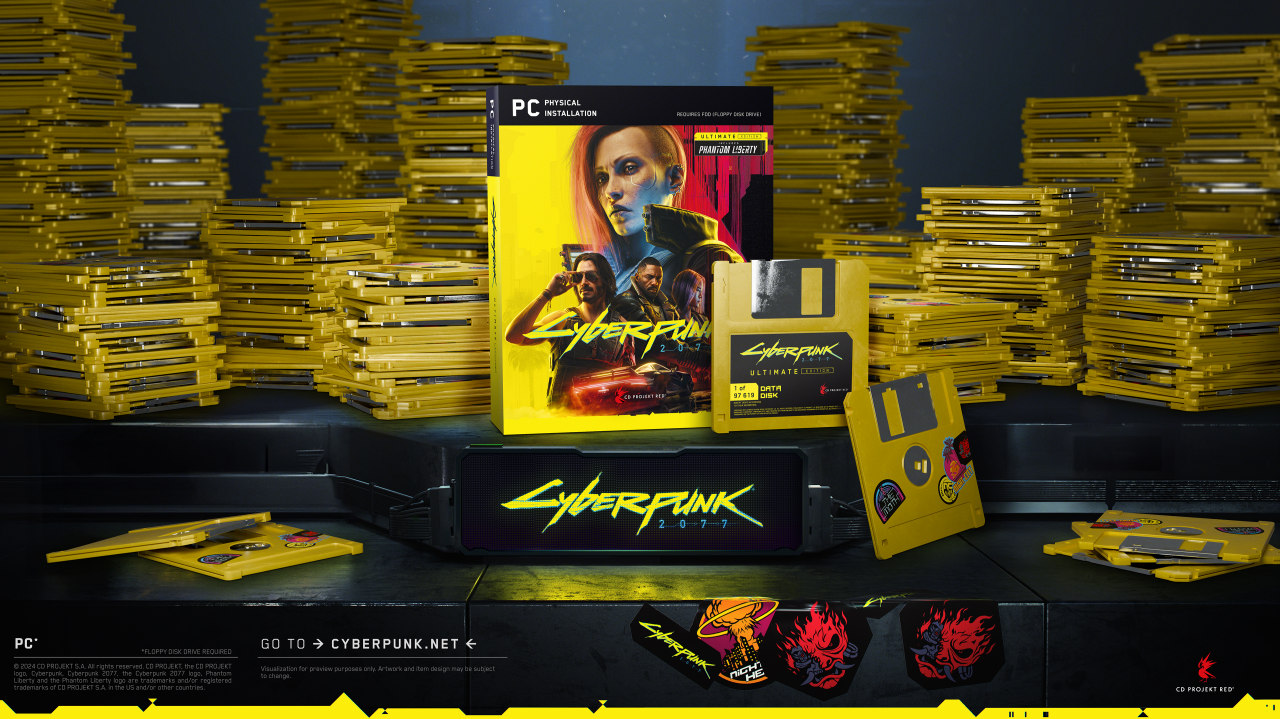The image depicts a nostalgic scene featuring hundreds of 3.5-inch yellow floppy disks meticulously stacked in the background, each with a distinctive silver metal circle in the middle and a rectangular cutout at the top for insertion into a computer drive. Dominating the center of the image is a prominently displayed black floppy disk with the bright yellow title "Cyberpunk 2077." Above this disk, a matching yellow cover reads "PC Physical Installation" in white text, with "Cyberpunk" beneath it in the same bright yellow font. The cover artwork features a dystopian collage of a girl's head, three men, and a red car, evoking a cyberpunk aesthetic reminiscent of the game’s themes. Additional stacks of floppy disks, varying in height, create a towering backdrop, all situated on a platform labeled "Cyberpunk." The scene captures the retro spirit of physical media, blending it with the futuristic allure of the Cyberpunk 2077 universe.